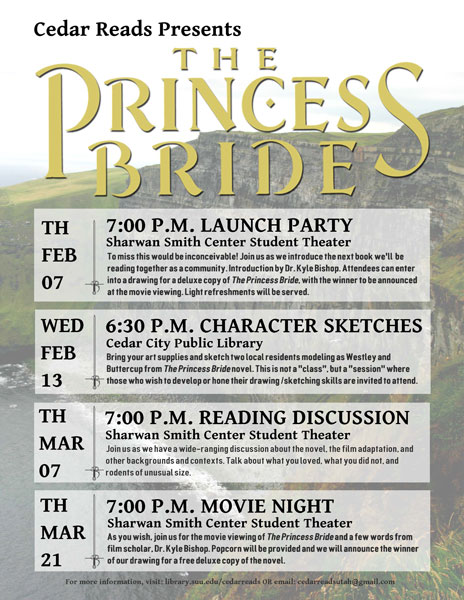The image appears to be an advertisement sheet for a series of events surrounding "The Princess Bride," presented by Cedar Reads. In the top left corner, it reads "Cedar Reads Presents" in black text. Below this, the title "The Princess Bride" is displayed in large, dark yellow, all-caps font, with a distinctive diamond shape inside the 'C' of "Princess." The background features a scenic hilltop or cliff with swings, and a body of water to the left.

Underneath the main title, there are four light gray text boxes, each with event details separated by small sword icons. The first box announces the launch party scheduled for Thursday, February 7th at 7 p.m. at the Charwon Smith Center Student Theater, featuring an introduction by Dr. Kyle Bishop. Attendees can enter a drawing for a deluxe copy of "The Princess Bride," with the winner announced at a later movie viewing. Light refreshments will be provided. 

The second box details a character sketches session on Wednesday, February 13th at 6:30 p.m. at the Cedar City Public Library. Participants are encouraged to bring their art supplies to sketch local residents modeling as characters Wesley and Buttercup.

The third box presents a reading discussion on Thursday, March 7th at 7 p.m. at the Charwon Smith Center Student Theater.

The final box promotes a movie night on Thursday, March 21st at 7 p.m., also at the Charwon Smith Center Student Theater, with popcorn provided. Below these boxes is more text, likely additional event details, but it is too small to read clearly in the image.